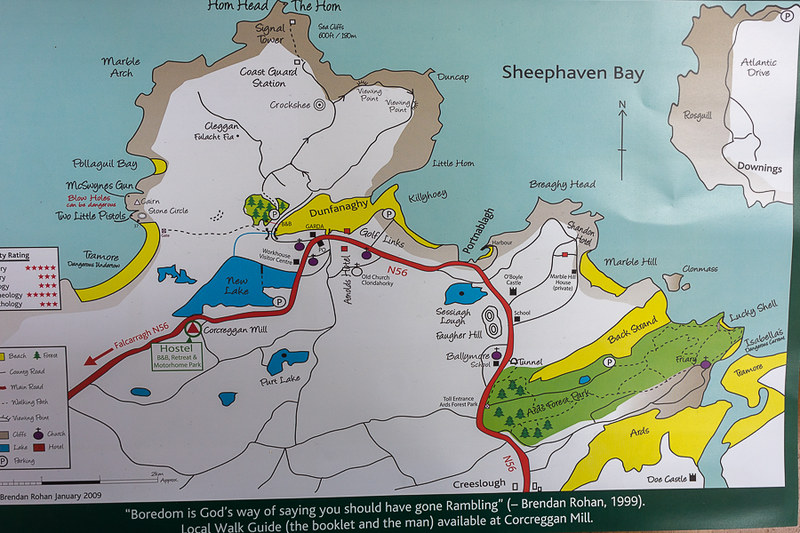This is a detailed color photograph of a map, likely depicting an area in Ireland given the names and locations shown. The map is bordered by a prominent green strip at the bottom, which includes a quote: "Boredom is God's way of saying you should have gone rambling," attributed to Brendan Rohan from 1999. Below the quote, it notes that this is a local walk guide available at Corcreggan Mill.

The map itself features a variety of geographically significant details. On the lower left side, there is a peninsula marked in white, dotted with blue lakes, green forests, and yellow sections labeled in black text. This area is bordered by a blue body of water, with Sheephaven Bay labeled in black text on the right side of the map. Additional notable areas include Marble Hill and Little Horn. The terrain is illustrated in varied colors including gray, blue, brown, and green, and a thin red line indicating a highway traverses the map. Also included is a legend positioned in the lower left-hand corner, albeit partially cropped. An arrow on the map indicates that north is up.